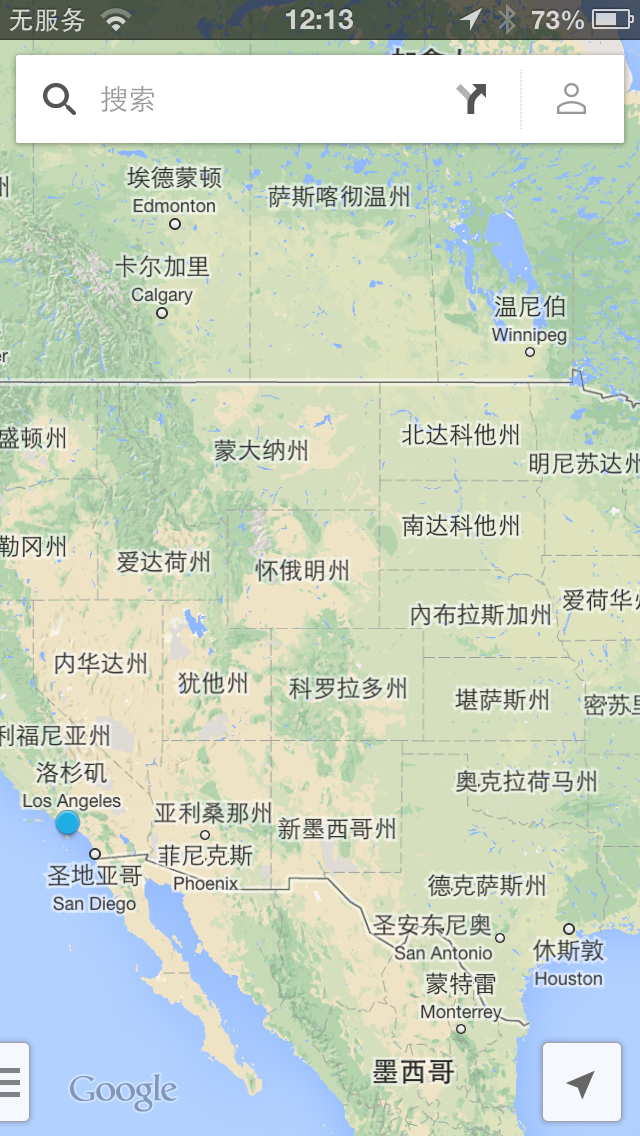This image is a screenshot of a smartphone screen displaying a geographical map of the Western United States, parts of Canada, and parts of Mexico. The map, predominantly rendered in light green with darker green denoting elevated areas, features place names primarily written in an Asian language, likely Chinese or Japanese. However, key city names are translated into English, including Los Angeles, San Diego, Phoenix, Houston, San Antonio, Monterey, Edmonton, Calgary, and Winnipeg. The map highlights natural features such as mountains, rivers, and lakes. The Google logo is visible in the lower left-hand corner. Also, the screenshot shows the device's status bar, indicating 73% battery power and the time as 12:13. The map extends from the West Coast, cutting off after Texas and includes some ocean at the bottom.